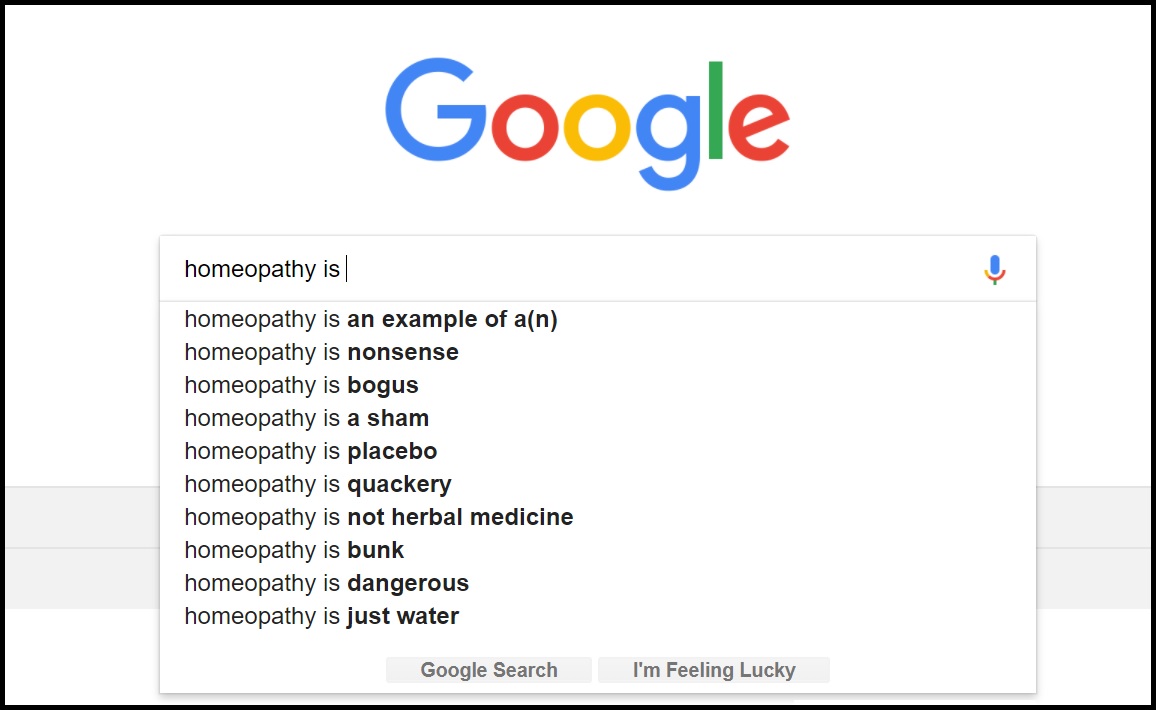The image features a search engine interface designed similarly to Google, but branded as "Gokli." At the top center of the image, the word "Gokli" is displayed using a colorful font: the first "G" is blue, the "O" is red, the second "O" is yellow, the second "G" is blue again, the "L" is green, and the "E" is red.

Below the brand name, there is a search box with a colorful microphone icon on its right side, adorned with Gokli's distinctive colors. Inside the search box, in white text, the phrase "homeopathy is" appears, indicating the beginning of a search query. A cursor is positioned at the end of this text, suggesting user interaction.

Under the search box, a list of autocomplete suggestions is displayed in descending order:
1. Homeopathy is an example of a N
2. Homeopathy is nonsense
3. Homeopathy is bogus
4. Homeopathy is a sham
5. Homeopathy is placebo
6. Homeopathy is quackery
7. Homeopathy is not herbal medicine
8. Homeopathy is bank
9. Homeopathy is dangerous
10. Homeopathy is just water

These suggestions, offered by Gokli, appear in a numbered vertical list format.

At the bottom of the image, there are two grey buttons with dark grey text. On the left is the "Gokli Search" button, and on the right is the "I'm Feeling Like" button. The entire image has a white background, maintaining a clean and minimalist aesthetic.